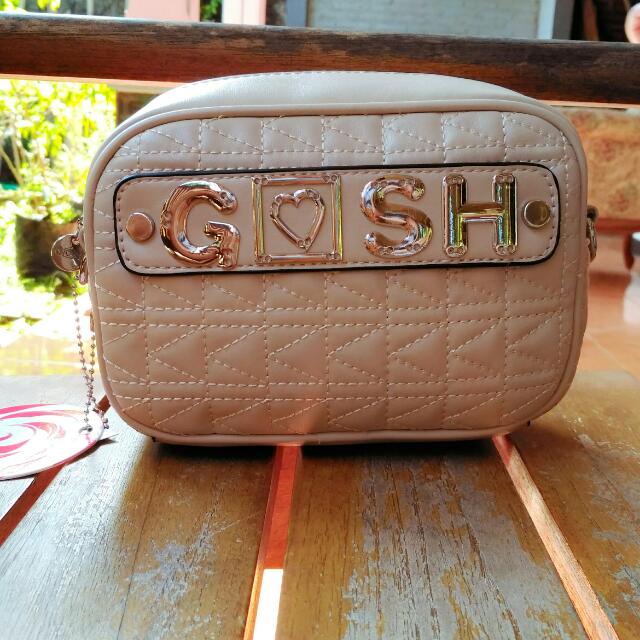This outdoor photograph captures a detailed close-up of a rectangular, tan-colored purse adorned with beige zigzag stitching. At the center of the purse, the word "GOSH" is prominently featured in gold letters, where the "O" is uniquely substituted with a heart inside a pink square. The letters are encased in a black rectangular bubble with rounded edges, secured to the purse with two circular pins on either side. The purse rests on a wooden surface, likely a bench or picnic table, identifiable by its vertical planks. Sunlight filters through the background, illuminating a ficus-like tree and a railing, suggesting the setting is a patio or garden. A CD lies to the left of the purse, adding to the scene's casual outdoor ambiance.